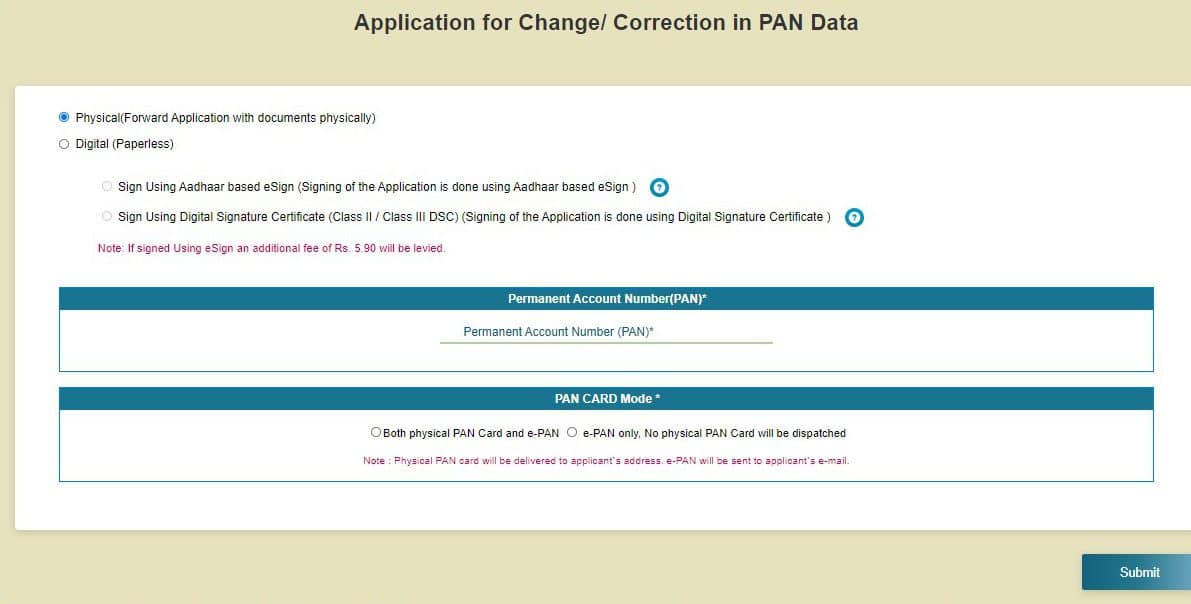Detailed Descriptive Caption:

The image illustrates an "Application for Change Correction to PAN" form interface. The primary background color is khaki, with a dominant white dialog box occupying about 80% of the screen's width, stretching expansively from left to right. This dialog box is split into sections for different application details.

At the top, the heading "Application for Change" is prominently highlighted in black. The form provides options for both physical and digital submissions, with interactive radio buttons for each selection. 

The first option reads "Physical" with a clickable dot currently highlighted in blue. Below this, the digital option labeled as "Paperless" in parentheses can be found, which includes a more indented sub-option: "Sign using Aadhaar-based e-sign." A question mark icon is positioned to the right of this text, offering additional information when clicked.

Another signing option follows, labeled "Sign using digital signature certificate, class 2/class 3."

Further down, an important note in pink text warns, "If signed using the e-sign, an additional fee of RS-590 will be levied."

The lower section of the form features a reverse-printed "Permanent Account Number (PAN)" heading, presented with white text on a blue background. Directly underneath, it restates "Permanent Account Number (PAN)" in standard font. Another reverse-printed section titles "PAN Card Mode," underneath which two selection options are available: "Both Physical PAN Card and e-PAN" and "e-PAN only." Accompanying this, a pink note informs that the "Physical PAN card will be delivered to the applicant's address."

Overall, the interface is designed for clarity, segregating physical and digital processes while providing clear instructions and additional information where necessary.